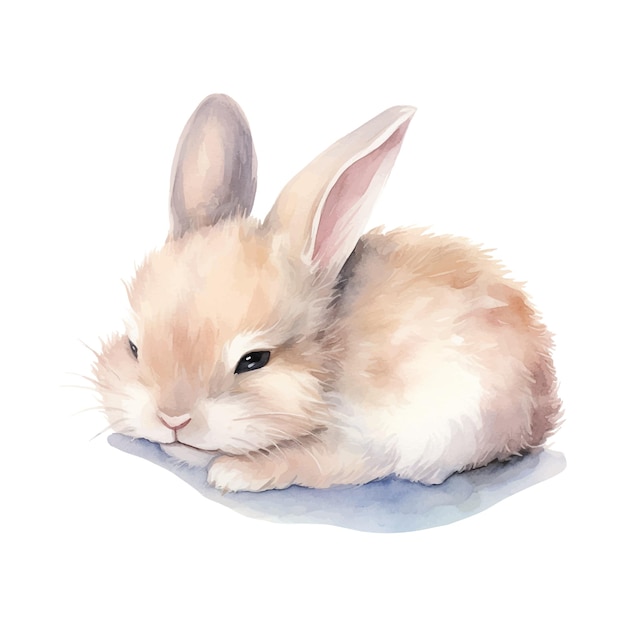This is a meticulously crafted illustration, likely a watercolor painting, of a baby rabbit. The bunny is very light brown with a soft, fluffy appearance and shades of cream, white, and pink. It lies on its stomach with its left arm tucked under its cheek, casting a shadow in dark blue beneath it. The ears are large with a pinkish hue on the inside, while the eyes are partially open, giving a drowsy, comfortable look. The rabbit's delicate whiskers are drawn in white, and it has a small, pink nose. The background is entirely white, creating a minimalistic and clean aesthetic that draws focus to the snuggly, relaxed bunny resting on what appears to be a small blue patch, possibly a blanket or some other surface.